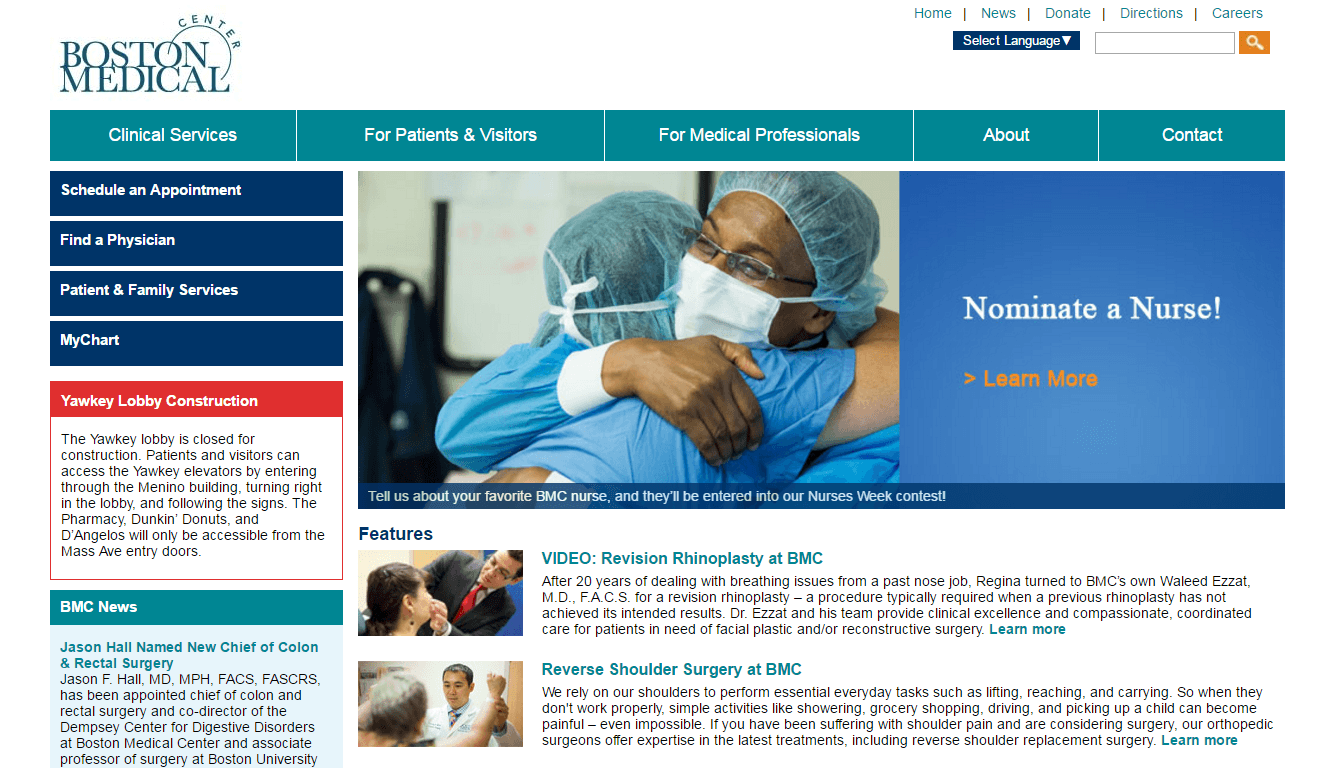This image captures the web page of Boston Medical Center in high detail. At the top left corner, the Boston Medical Center logo is prominently displayed. The logo features the words "Boston" and "Medical" stacked in two lines. "Boston" is written in green letters, and a thin circle begins from the 'O' and curves down to the 'L' in "Medical," with "Center" positioned near the top of the circle.

The navigation panel across the top includes five menu choices, each delineated by thin white lines yet connected by green buttons. The options are: "Clinical Services," "Patients & Visitors," "For Medical Professionals," "About," and "Contact." 

Below this, there is a compelling photo of two nurses embracing. One nurse, whose face is visible, is wearing a mask over her mouth and nose and a pair of glasses. Both nurses are dressed in medical attire, indicating their professional bond.

To the right of this image, a blue box with bold white text stands out, encouraging visitors to "Nominate A Nurse!" with an exclamation point. A "Learn More" button is placed below this call to action.

Further down, aligned horizontally, are four dark blue boxes with white writing, labelled as follows from top to bottom: "Schedule An Appointment," "Find A Physician," "Patient and Family Services," and "My Chart."

Beneath the touching image of the nurses, there are two linked video thumbnails. The first video is titled "Revision Rhinoplasty at BMC." Adjacent to the title is a thumbnail featuring a doctor, dressed in a suit and tie, examining a patient. The video description follows underneath.

The second video is titled "Reverse Shoulder Surgery at BMC," showcasing a doctor examining what seems to be an older woman. A detailed description accompanies the title below the thumbnail.

To the left of these sections, there's a box labelled "Yawkey Lobby Construction" and another one marked "BMC News." Under the "BMC News" headline, the singular brief item announces "Jason Hall Named New Chief of Colon and Rectal Surgery."

The web page layout effectively organizes critical information, helping visitors navigate the content seamlessly while providing vital updates and features from Boston Medical Center.